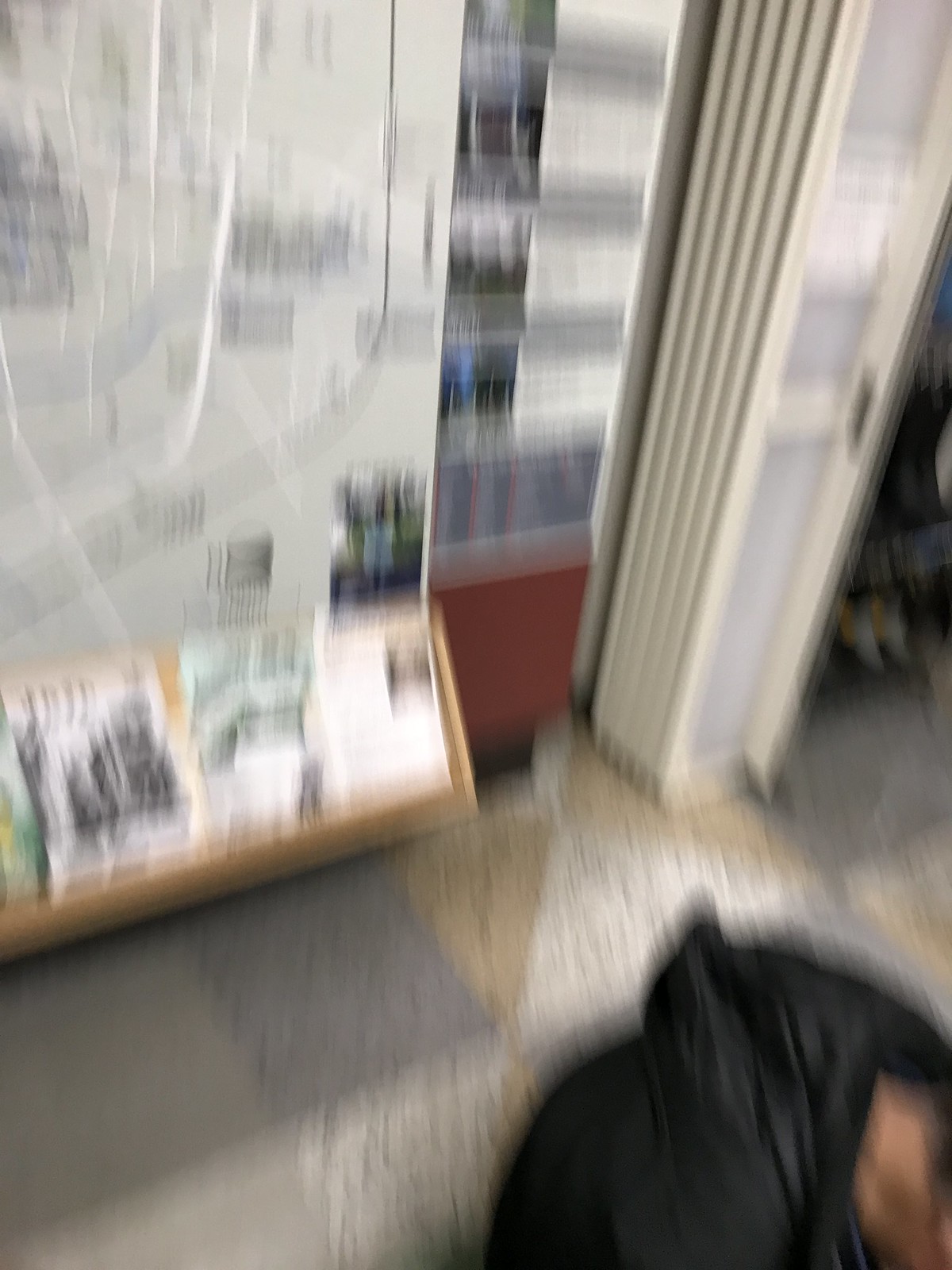A blurry and slightly out-of-focus photograph captures a scene within a room. Dominating the background is a large map affixed to the wall, accompanied by a light brown wooden shelf below it. The shelf appears to hold various papers, potentially flyers or real estate images. In the foreground sits a person dressed in a black raincoat with the hood up, sitting on a tiled floor of gray, white, and tan hues. A small portion of their reddish-pinkish neck is visible to the right. Adjacent to the map on the right is a narrow, bifold door, currently closed, with an accordion-style design. The overall composition suggests a somewhat cluttered yet informative environment.